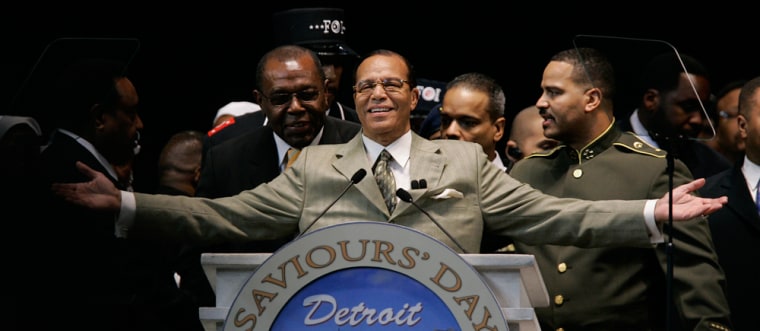This image captures a significant moment featuring Minister Louis Farrakhan of the Nation of Islam during the Savior's Day event in Detroit. The horizontal, rectangular photo presents a scene set against a dark background, with the top of a sign in front of the podium reading "Savior's Day" and "Detroit" in white letters on a blue field. Minister Farrakhan stands at the podium, which is equipped with two microphones. He is wearing a light tan or gray suit, complemented by a white button-down shirt and a brown and tan tie. A handkerchief is visible in his breast pocket, and he is smiling as he addresses the audience with his hands outstretched, palms facing upward.

Surrounding Minister Farrakhan are several men, all appearing to have short hair and wearing suits, with one man in a green military-style uniform with gold buttons positioned to his right. Behind him, two men wearing dark uniforms and F.O.I. (Fruit of Islam) caps can be seen, underscoring the presence of the Nation of Islam's security force. The light source above Minister Farrakhan adds emphasis to the scene, highlighting his central role in this moment of communal celebration and support.